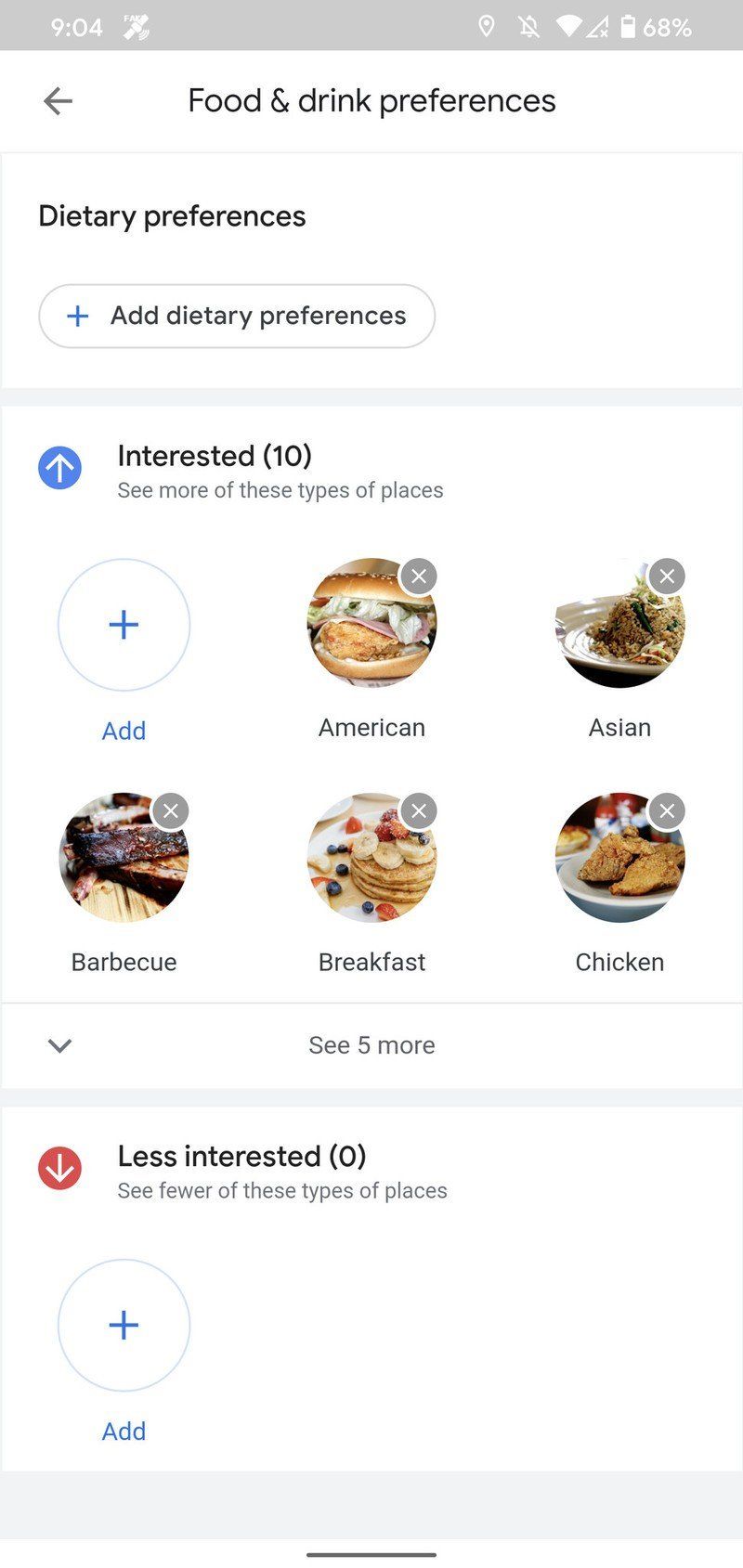The screenshot displayed on a phone captures various interface elements and app features. In the top left-hand corner, the time is shown as 9:04, alongside a small plane icon, which is likely associated with a travel app. On the right side of the top bar, a series of icons are visible: a location services icon resembling a bubble, a bell icon with a dash through it indicating the phone is on silent mode, a Wi-Fi signal icon, a triangle icon (potentially cellular data), and finally, a battery icon with a remaining charge of 68%.

Below this top toolbar, the screen displays a section titled "Food and Drink Preferences," accompanied by a leftward arrow icon. Beneath this title, there is a subsection labeled "Dietary Preferences" which includes an option to "Add Dietary Preferences" with a plus button for user interaction.

The next panel features an "Interested" section with an upward arrow and the number 10 in parentheses, followed by the text "See more types of these places." On the left side of this panel, there is a blue circle with a plus sign, indicative of an option to add more interests. To the right are categorized food preferences: an image of a burger labeled "American Food," an image of Asian cuisine titled "Asian Food," an image of barbecue labeled "Barbecue," an image of pancakes labeled "Breakfast," and a picture of chicken labeled "Chicken." 

Underneath these, an arrow pointing downwards invites the user to "See five more" preferences. The following section labeled "Less Interested" features a downward arrow, a red color scheme, and the number 0 in parentheses, inviting users to indicate fewer preferences and "See fewer of these types of places."

At the very bottom of the screen, there is another blue circle with a plus sign, providing an option for users to add additional entries or preferences.